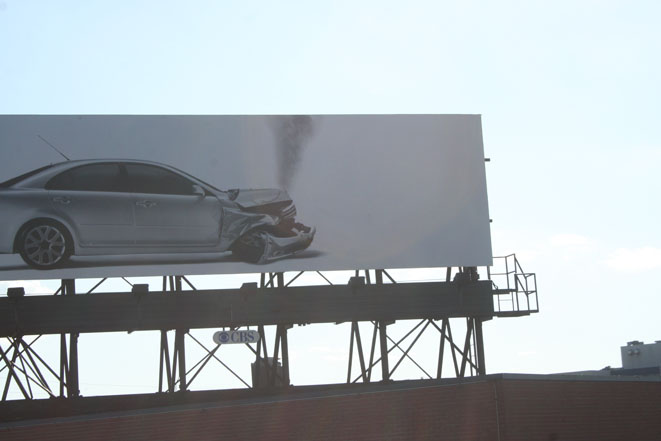A detailed, cleaned-up description of the image could be:

"The image captures a billboard mounted atop a red brick building, photographed during daylight under a pale blue sky with a faint cloud to the right of the billboard. The billboard itself features a stark white background showcasing a gray vehicle that appears to have been in a severe accident. The car's front end is demolished, with visible smoke billowing from under the crumpled hood, a detached bumper, and a displaced front right tire. The car's windows are tinted, adding to the dramatic effect of the wreckage. Beneath the billboard, an eyeball and the acronym 'CPS' are prominently displayed, likely part of the advertisement's message."